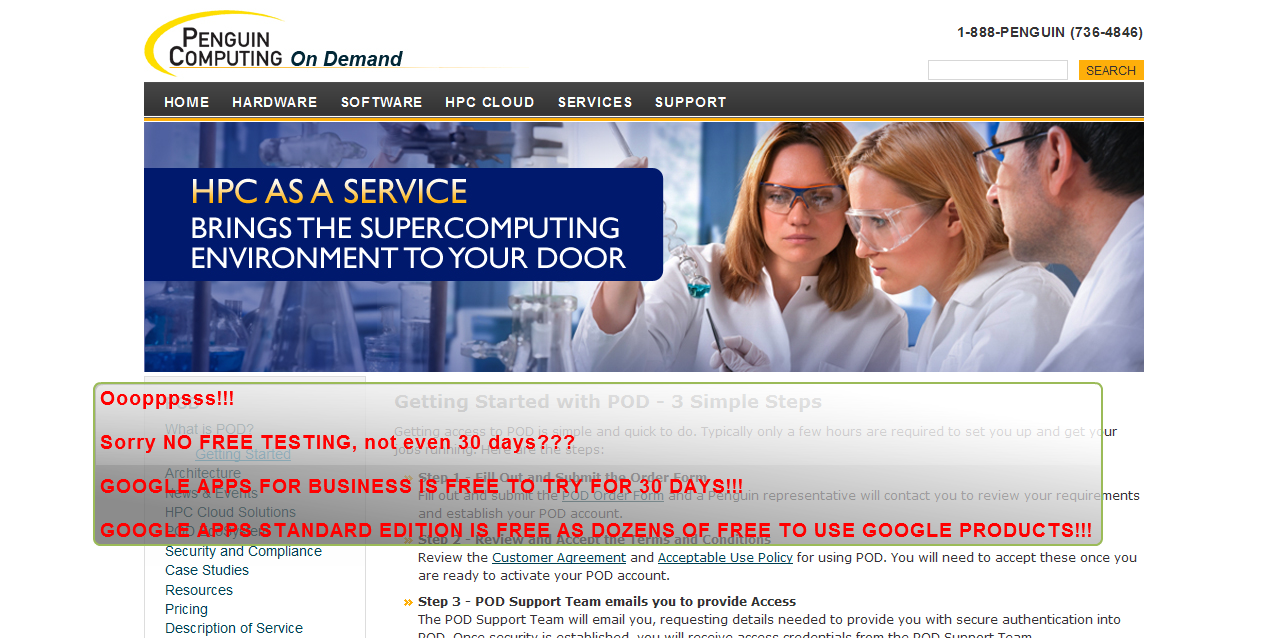The image is a detailed screenshot of a website landing page for "Penguin Computing On Demand", prominently featuring the logo with a yellow semi-circle around black text in the upper left corner. The top navigation menu, against a gray background, includes links to Home, Hardware, Software, HPC, Cloud, Services, and Support, with the phone number 181-888-PENGUIN displayed in the upper right. The main visual is a full-color photograph of three scientists or doctors, two women and one man, all dressed in white lab coats and safety goggles, handling chemicals. The header text reads "HPC as a service brings the supercomputing environment to your door". Superimposed on the image is red text in a gray block stating, "Oops!!! Sorry, no free testing. Not even 30 days??? Google Apps for Business is free to try for 30 days. Google Apps Standard Edition is free as dozens of free to use Google products." Below this, a couple of paragraphs titled "Getting Started with POD" are visible at the bottom of the image. The background predominantly features blue shades, adding a professional and sleek touch to the layout.